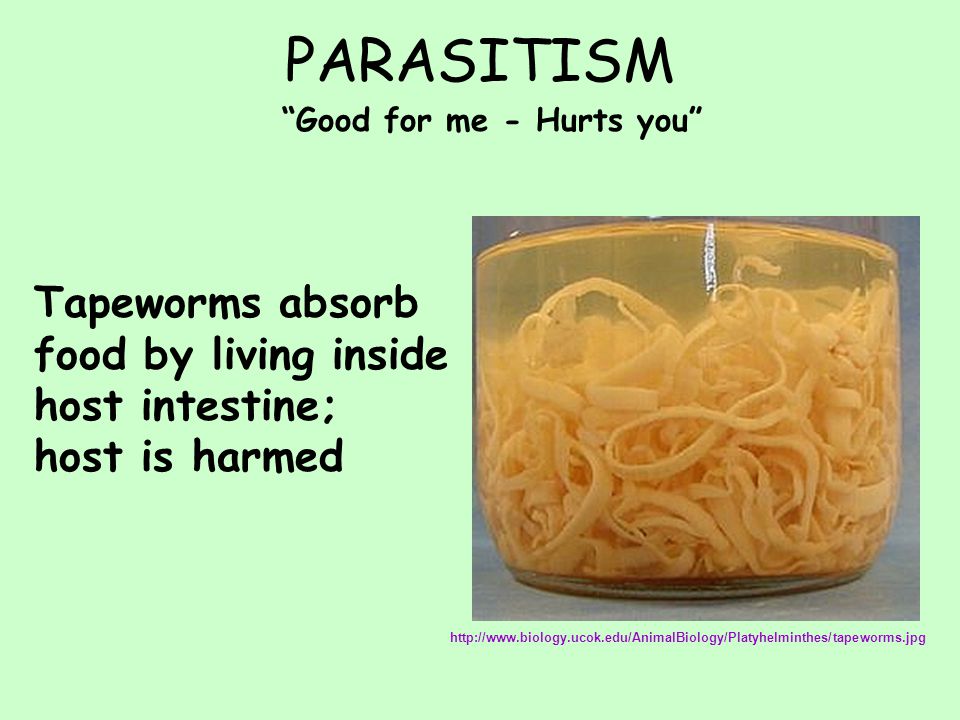The image is an educational slide designed in a nearly square, light mint green (or lime green) background, likely from a PowerPoint presentation. At the top center, large black uppercase text reads "PARASITISM," and just below it, a smaller black text in quotation marks states, "good for me - hurts you." To the left center, the slide features black Comic Sans text explaining: "Tapeworms absorb food by living inside host intestine; host is harmed," with the T in "Tapeworms" capitalized.

To the right of this explanatory text, there is a square image with a purple background. The image depicts a large round plastic or glass container filled almost to the brim with what appears to be numerous beige, noodle-like tapeworms, reminiscent of light yellow fettuccine. Beneath the image, a URL is provided in small purple Arial font: "http://www.biology.ucok.edu/animal_biology/platyhelminthes/tapeworms.jpg."